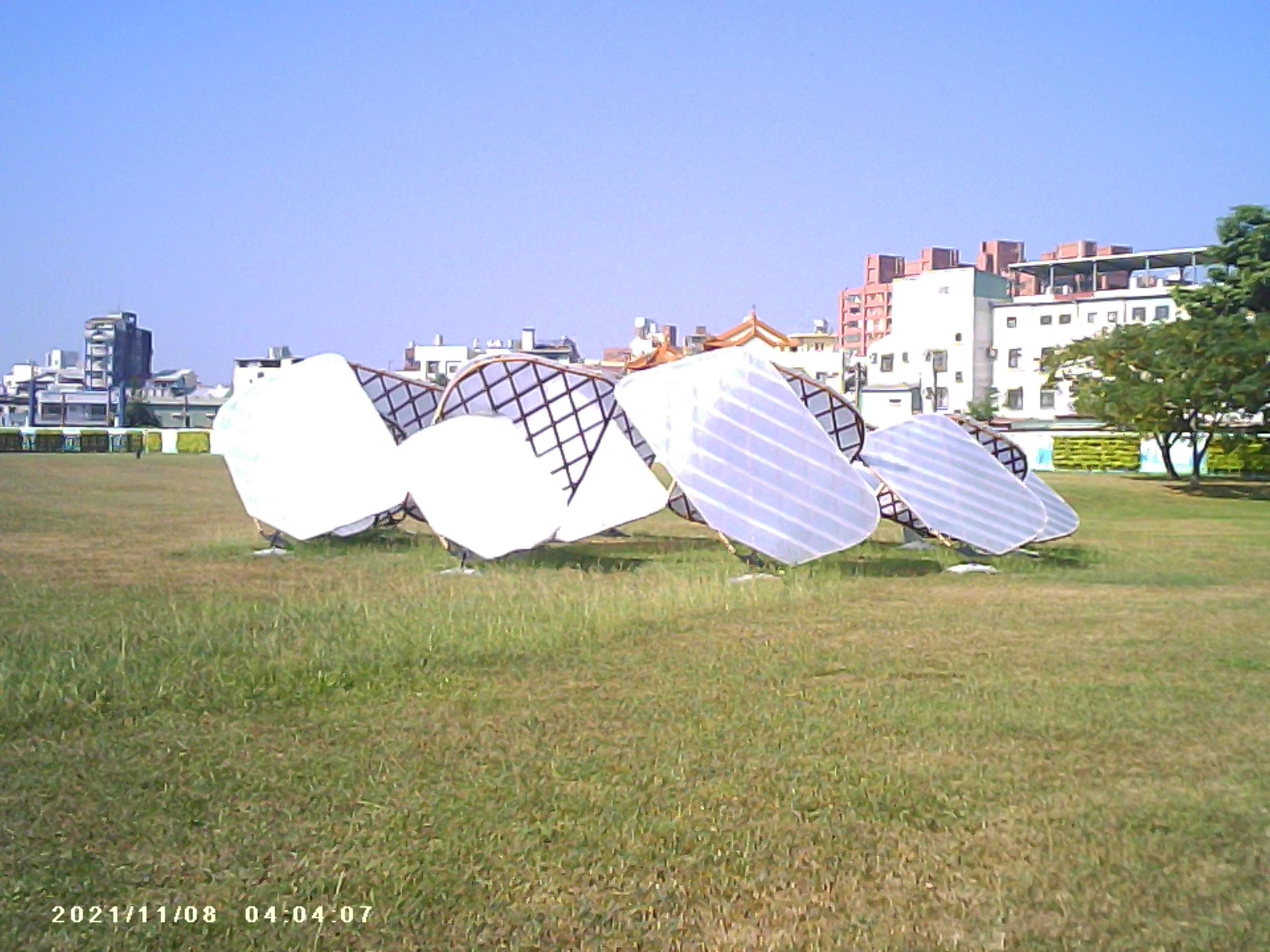In this image, we observe a bright, sunny day in a wide-open, grassy space, likely part of a park. The lush green field, interspersed with patches of brown, extends outward to the right where a tree stands and possibly some benches can be discerned. Dominating the background is a highly metropolitan area featuring large buildings that appear to be hotels or factories, with some more indistinct buildings to the left. The sky is a pristine blue, devoid of any clouds. In the foreground, at the center of the image, a collection of silver solar panels with black lines are arranged at varying angles. These panels come in different shapes, including a lemon, a triangle, a square, and a rectangle. Some of the panels have reflective white highlights, with portions washed out by the sun. Additionally, there's a brown diamond mesh structure among the solar panels. The bottom left corner of the image displays a timestamp: November 8th, 2021, at 4:04:07 PM.